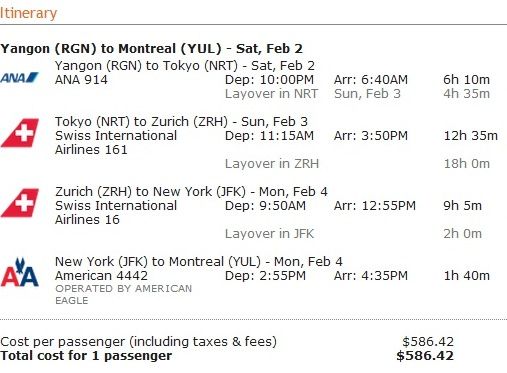**Travel Itinerary Overview:**

**Flight Details:**

***Yangon (RGN) to Montreal (YUL)***

**Date**: Saturday, February 2nd

**Airline**: ANA

1. **First Leg:**
   - **Route**: Yangon (RGN) to Tokyo (NRT)
   - **Flight Number**: ANA 914
   - **Departure Time**: 10:00 PM
   - **Arrival Time**: 6:40 PM (Sunday, February 3rd)
   - **Duration**: 6 hours 10 minutes

2. **Layover in Tokyo (NRT)**:
   - **Duration**: 4 hours 35 minutes

**Continuing Onward:**

***Tokyo (NRT) to Zurich (ZRH)***
   
**Airline**: Swiss International Airlines 

1. **Second Leg:**
   - **Route**: Tokyo (NRT) to Zurich (ZRH)
   - **Flight Number**: SWISS International Airlines 161
   - **Departure Time**: 11:15 AM (Sunday, February 3rd)
   - **Arrival Time**: 3:50 PM
   - **Duration**: 12 hours 35 minutes

2. **Layover in Zurich (ZRH)**:
   - **Duration**: 18 hours

**Next Segment:**

***Zurich (ZRH) to New York (JFK)***

**Airline**: Swiss International Airlines
   
1. **Third Leg:**
   - **Route**: Zurich (ZRH) to New York (JFK)
   - **Flight Number**: SWISS International Airlines 16
   - **Departure Time**: 9:50 AM (Monday, February 4th)
   - **Arrival Time**: 12:55 PM
   - **Duration**: 9 hours 5 minutes

2. **Layover in New York (JFK)**:
   - **Duration**: 2 hours 

**Final Segment:**

***New York (JFK) to Montreal (YUL)***

**Airline**: American Airlines, operated by American Eagle

1. **Fourth Leg:**
   - **Route**: New York (JFK) to Montreal (YUL)
   - **Flight Number**: American Airlines 4442
   - **Departure Time**: 2:55 PM
   - **Arrival Time**: 4:35 PM
   - **Duration**: 1 hour 40 minutes

**Cost Information:**
- **Cost per Passenger (Including Taxes and Fees):** $586.42
- **Total Cost for One Passenger:** $586.42

This covers the comprehensive travel route from Yangon to Montreal with specific details on flight numbers, layovers, and durations for a clear understanding of the journey.